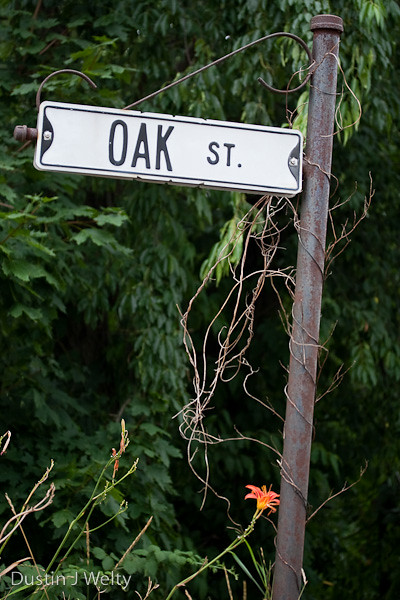The photograph captures a rustic street sign mounted on a weathered, copper-hued pole entwined with twisting branches or vine-like structures. The sign itself is suspended from a brass hanger that extends to the left side of the pole. It features a white background with dark gray-black lettering that reads "Oak Street," followed by a period. The backdrop consists of a lush natural scene, with vibrant green foliage and a single orangey-red flower emerging from the bottom of the image. The scene is devoid of any residential structures, focusing solely on the sign and its surroundings. In the bottom left-hand corner, the name "Dustin J. Welty," presumably the photographer, is inscribed.